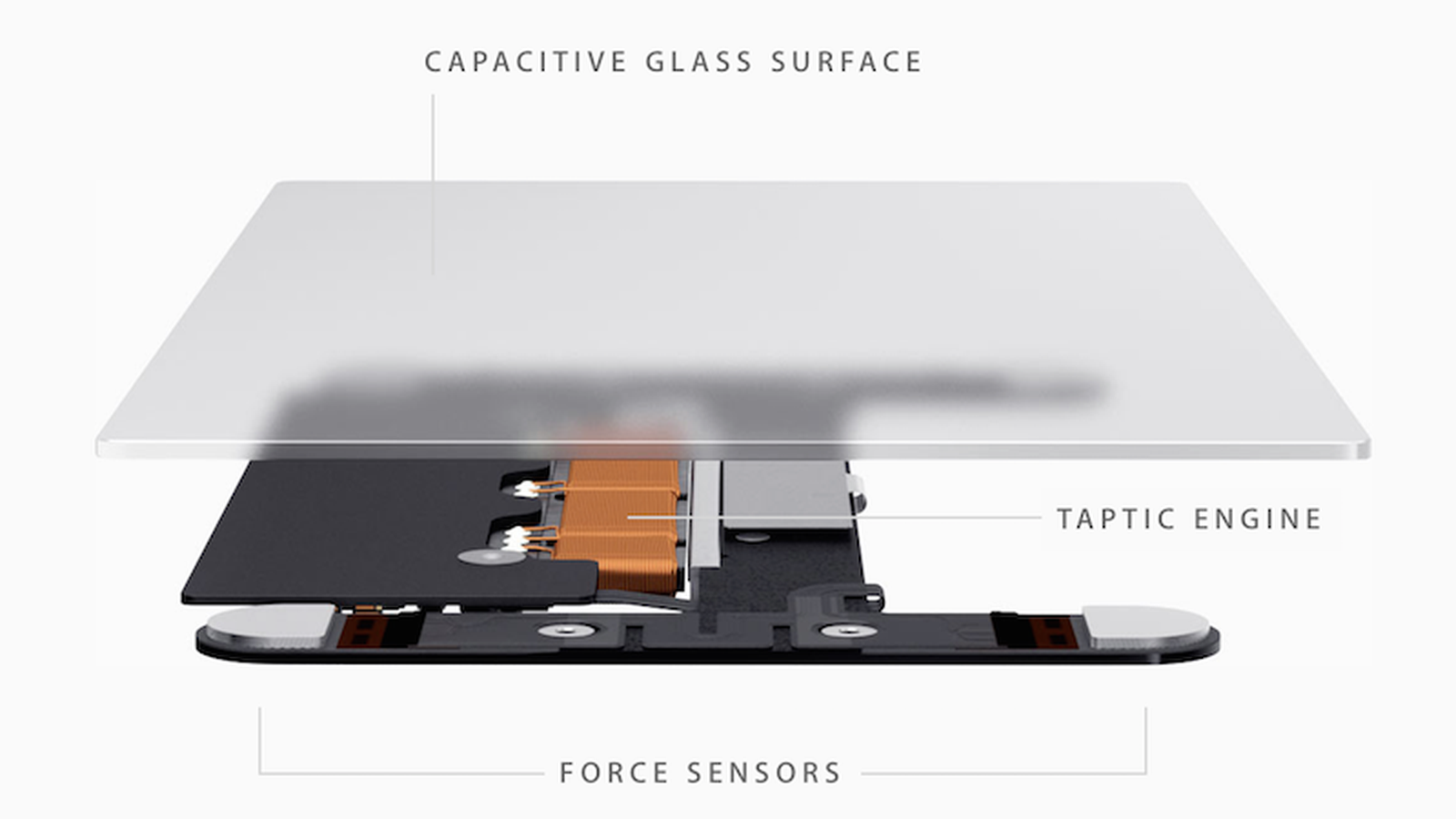This photorealistic diagram, though not a photograph, showcases a disassembled electronic gadget in a landscape orientation. At the top, there's a rectangular grayish frosted glass panel labeled "Capacitive Glass Surface." Just beneath this glass piece lies the complex inner workings of the device, predominantly highlighting the "Taptic Engine." This component features prominent copper-colored coils at its center, surrounded by a black structure that resembles a flat holder or DVD tray. Below the Taptic Engine, the "Force Sensors" are indicated, represented as small, black foot pad-like elements, extending out with metal tips. Additionally, there are silver nuts and bolts visible around the base, lending further detail to the intricate assembly of this electronic product.